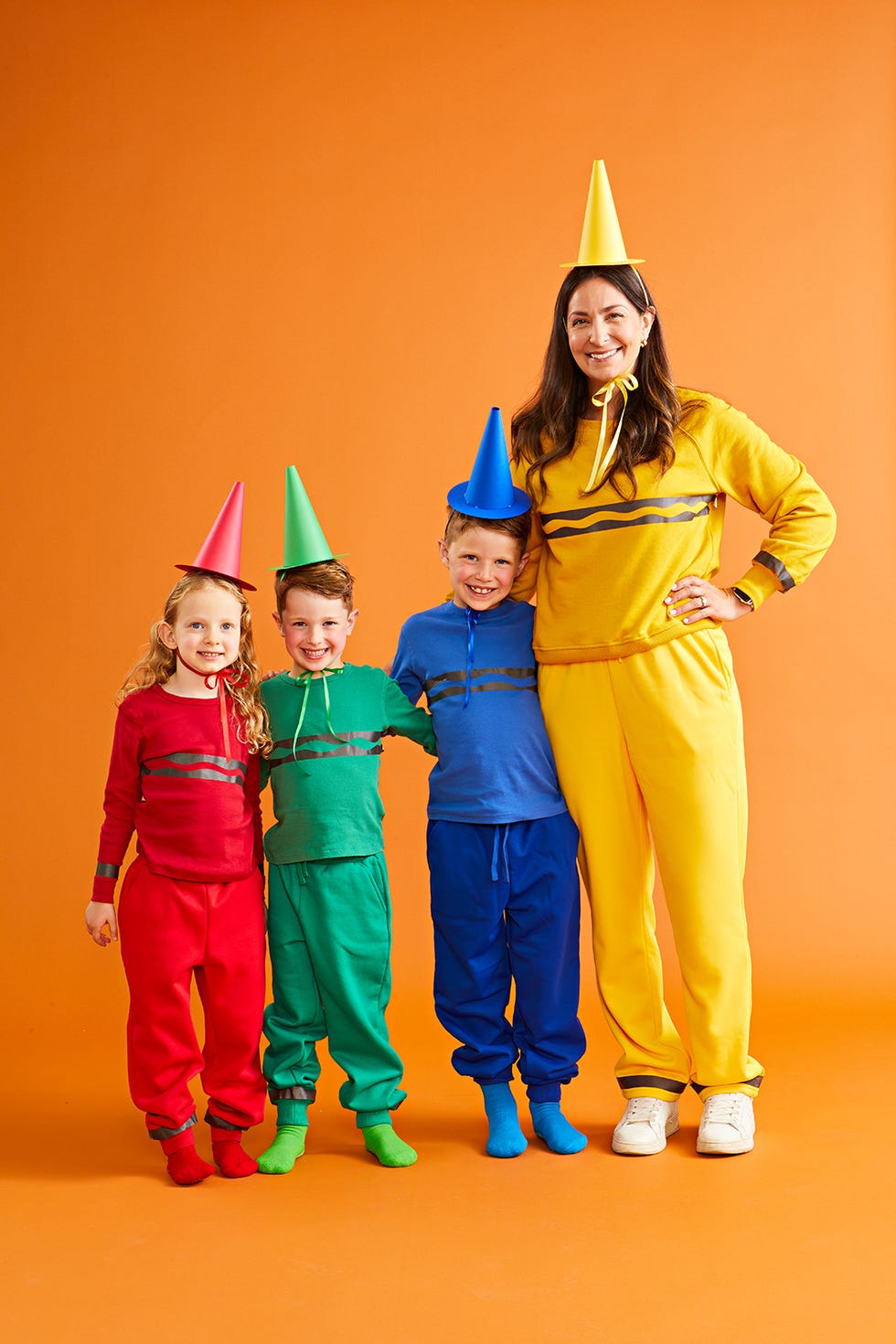In a vibrant and playful photography setting, this engaging portrait features a woman and three children, all joyfully dressed as crayons. The floor and backdrop seamlessly merge into a bright orange expanse, creating a warm, cheerful atmosphere. The woman, appearing to be the mother, is adorned in a full yellow crayon outfit, complete with a shirt bearing the classic black crayon mark and a pointed hat mimicking a crayon tip. She stands with one hand placed confidently on her hip and the other lovingly around a boy in a blue crayon suit. The children, undoubtedly siblings, exhibit a colorful array of crayon costumes: the girl in red with blonde hair and matching socks, a boy in green with brown hair, and another boy in blue, wrapping an arm around the child in green. Each child is meticulously dressed head-to-toe in their respective crayon color, right down to their socks, while the woman sports white shoes. All four figures are united in a close embrace, beaming with radiant smiles as they gaze directly into the camera, capturing a moment of pure, joyful togetherness.